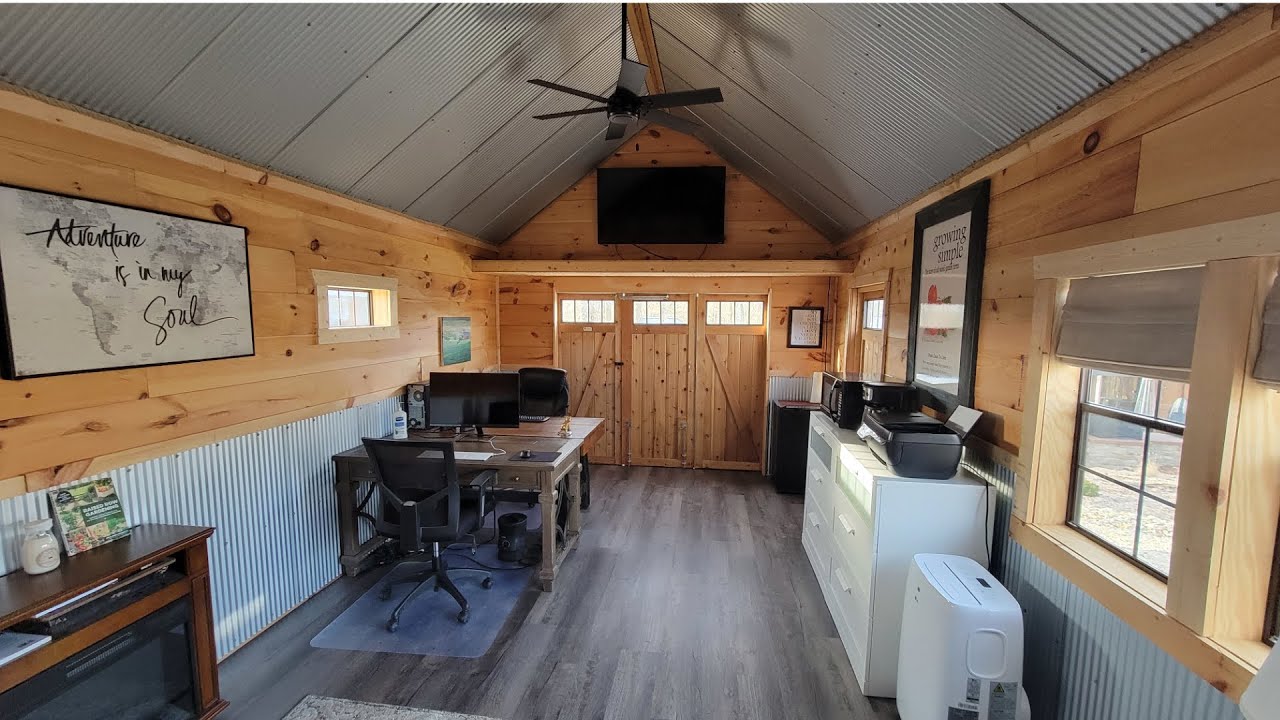The photograph depicts the interior of a transformed barn, now serving as a cozy home office. The structure boasts a galvanized steel roof with a corrugated silver finish, complemented by light and dark brown wooden paneling throughout, creating a warm, rustic atmosphere. The A-frame ceiling, adorned with a basic black ceiling fan, converges at the center, accentuating the barn's traditional architecture. The wooden floor is a rich, dark brown, extending across the space.

Two desks are set up against the walls, each equipped with chairs and a monitor. One desk also houses a printer, while a white dresser nearby holds a microwave and a coffee machine, emphasizing the space's functionality as a work area. The office decor is simple yet classic, featuring a limited color palette of browns, whites, and silvers.

On the left wall, a picture of a map with the words "Adventure is in my soul" exudes inspiration, hanging above an electric fireplace that adds a touch of warmth. Toward the far end of the room, three barn-style doors with long rectangular windows introduce additional natural light. Situated within the cozy office are a TV mounted on the wall and a white table, providing a versatile area for meetings or breaks. This idyllic setup combines the charm of rustic design with the practicalities of a modern home office.